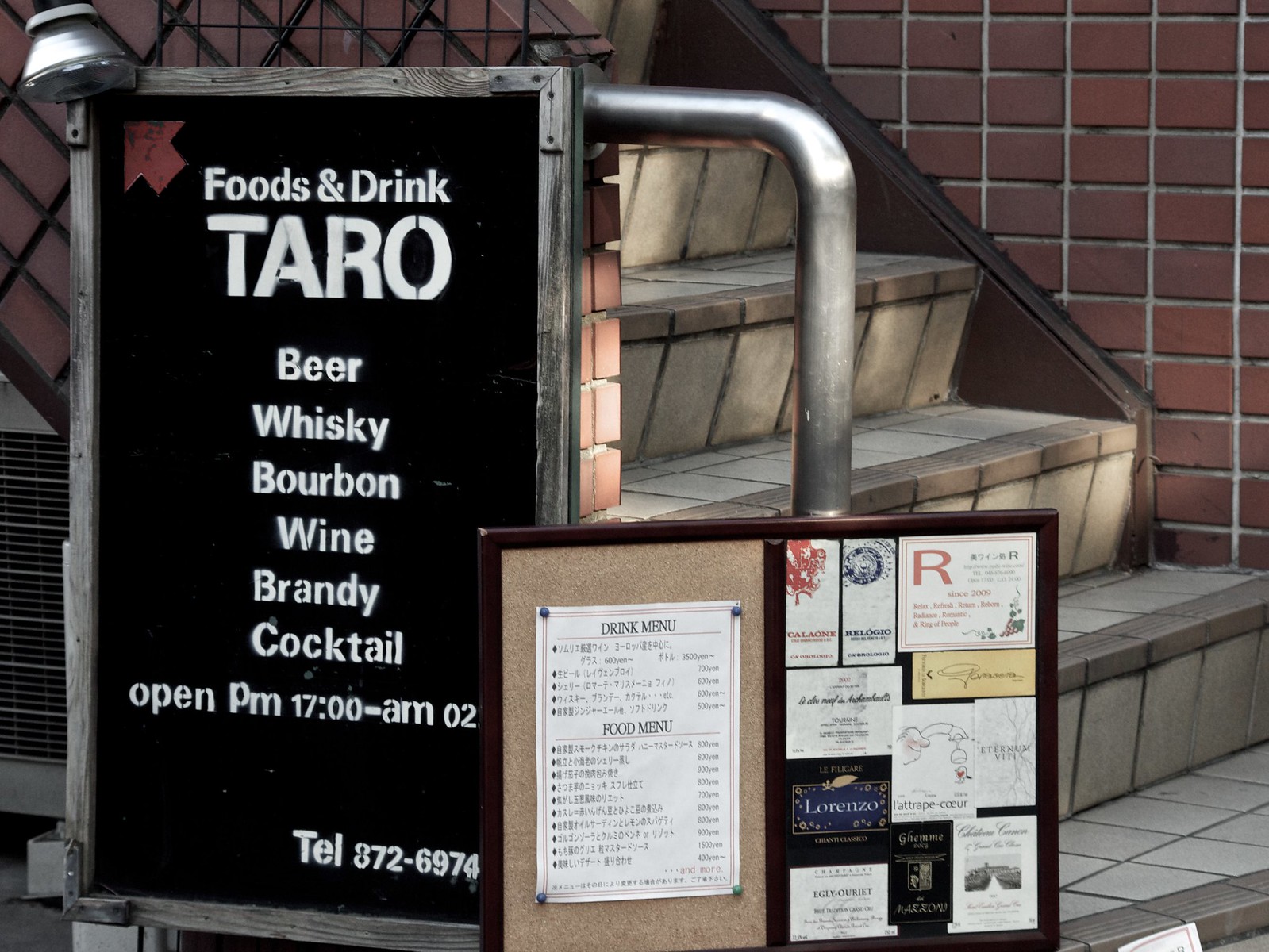The image captures a close-up view of a staircase leading to what appears to be a restaurant or bar. The stairs, adorned with brown and cream-colored tiles, ascend from the lower right to the top middle of the picture, flanked on the right by a silver metal handrail and a red brick wall. On the left side of the image is a prominently displayed sign within a wooden frame, featuring a black background with white font that reads: "Foods and Drink, Taro (T-A-R-O), beer, whiskey, bourbon, wine, brandy, cocktail. Open p.m. 1700 to a.m. 0200." A telephone number, 872-6974, is listed at the bottom right of the sign. Adjacent to this is a cork board with several papers pinned, including a detailed drink and food menu. The setting exudes the ambiance of a possibly older bar or restaurant in a grungier building, inviting patrons with its rustic and intimate charm.